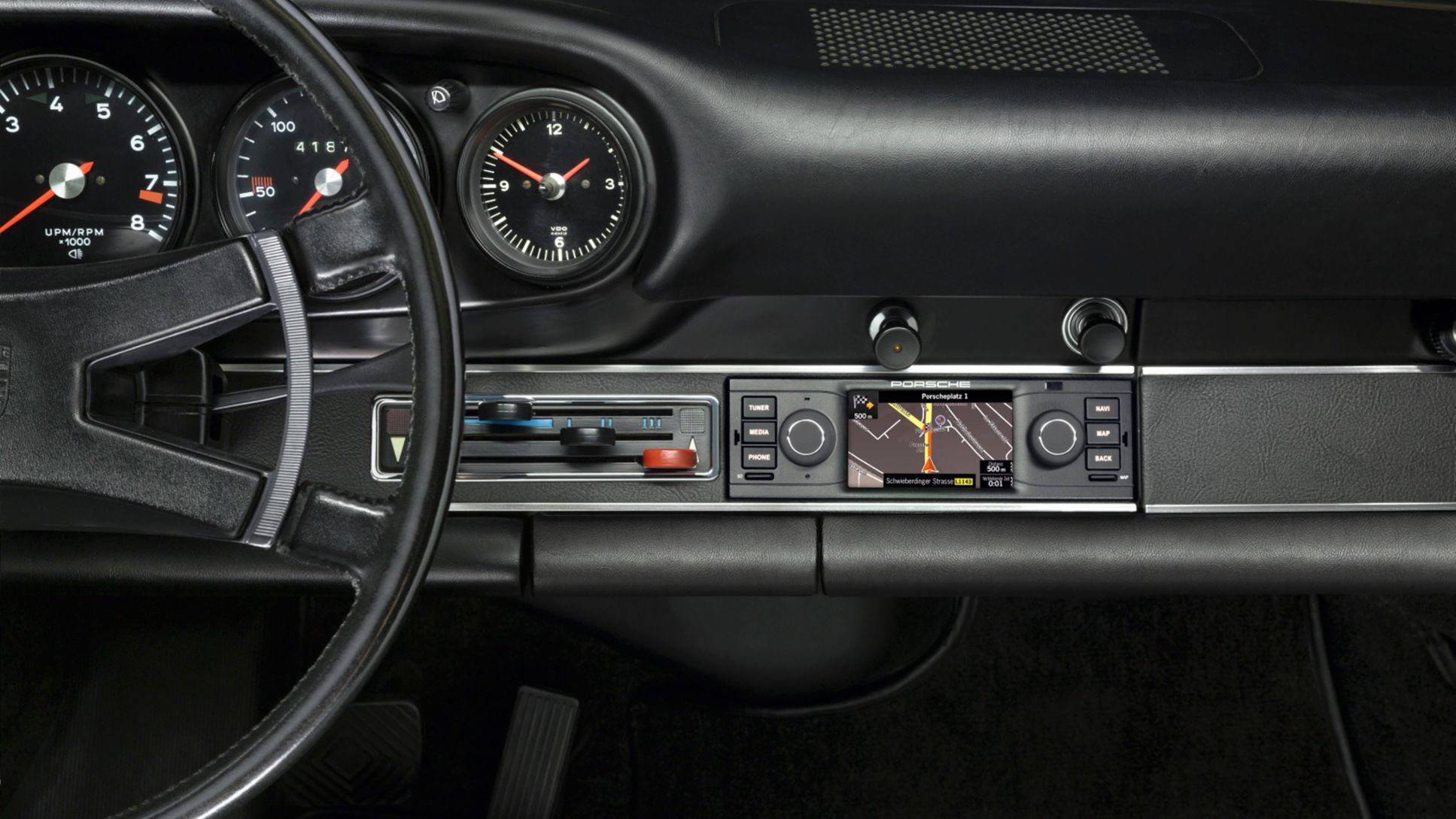This photograph captures the detailed interior of a car's dashboard, predominantly black with a vinyl finish, complemented by a modern GPS system. The left side features part of a black steering wheel, and behind it, the dashboard displays three circular dials: a tachometer reaching 8,000 RPM on the far left, a speedometer with visible markings at 50 and 100 kilometers per hour in the center, and a clock showing ten minutes to 2 o'clock on the far right. Below these, the dashboard includes black and red knobs for heater and air conditioner controls, alongside sliders reminiscent of older car models.

To the right, the GPS device with a backlit LCD screen illustrates a street and highlighted route in yellow and red. Flanking the screen are two knobs, with three vertical rows of buttons on each side. Further below, a modern USB port appliance replaces the traditional cigarette lighter, enhancing the blend of vintage and contemporary elements in this car. The carpet, brake pad, and accelerator visible at the bottom add to the all-black aesthetic, offset only by the contrasting colors used in the gauges and controls. This blend of modern equipment within a classic layout suggests a newer vehicle designed with a retro appeal.